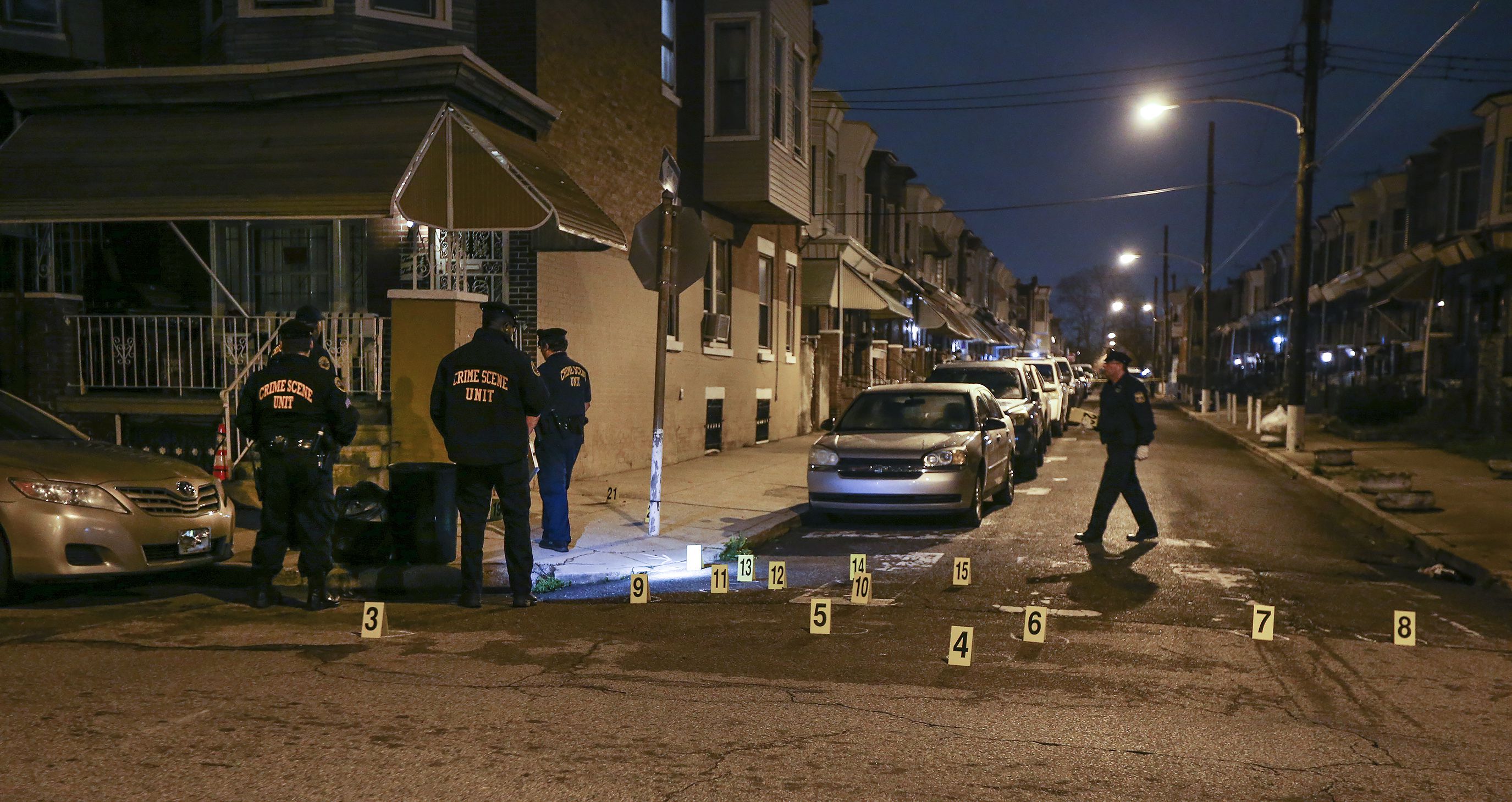The nighttime photograph captures a crime scene on a residential street corner, illuminated by streetlights and accented by the occasional house lights in the distance. The scene is cordoned off, with multiple cars parked along the curbs and light posts scattered throughout the area. Four police officers, dressed in black uniforms — one of whom is crossing the street — are focused on the scene. Their jackets read "Crime Scene Unit." The officers appear to be examining a spotlighted area on the corner, where a wet substance is visible on the ground. Scattered across the street and sidewalk are numerous evidence markers, numbered sequentially from 1 to at least 15. Additional details include trash cans near the crime scene and a house with a staircase and balcony that seemingly attracts the officers' attention.